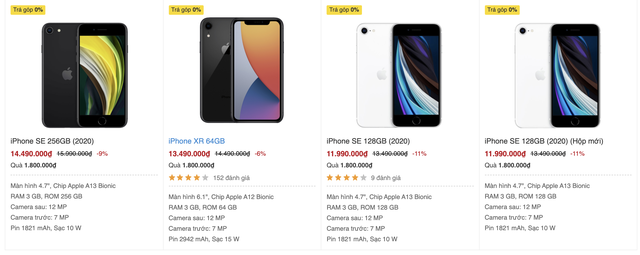The image features four iPhones displayed for sale, each showcased with their front and back views. The distinct Apple logo is visible on the back of each device. The screens of the iPhones feature colorful, vibrant wallpapers. Below is a detailed description of each iPhone:

1. **iPhone SE (2020)**: 
   - **Storage**: 64 GB
   - **Condition**:  Originally priced at an unclear amount 
   - **Discount**: 9% off
   
2. **iPhone XR**: 
   - **Storage**: 64 GB
   - **Condition**: Shows a rating of 4 to 5 stars
   - **Discount**: 6% off

3. **iPhone SE (2020)**:
   - **Storage**: 128 GB
   - **Condition**: Also rated between 4 to 5 stars
   - **Discount**: 11% off

4. **iPhone SE (another 2020 model)**:
   - **Storage**: 128 GB
   - **Condition**: Mentioned as "Hopmon" although the meaning is unclear
   - **Discount**: 11% off

All four iPhones have experienced a price reduction, though the exact original and current prices are not clearly visible in the image.